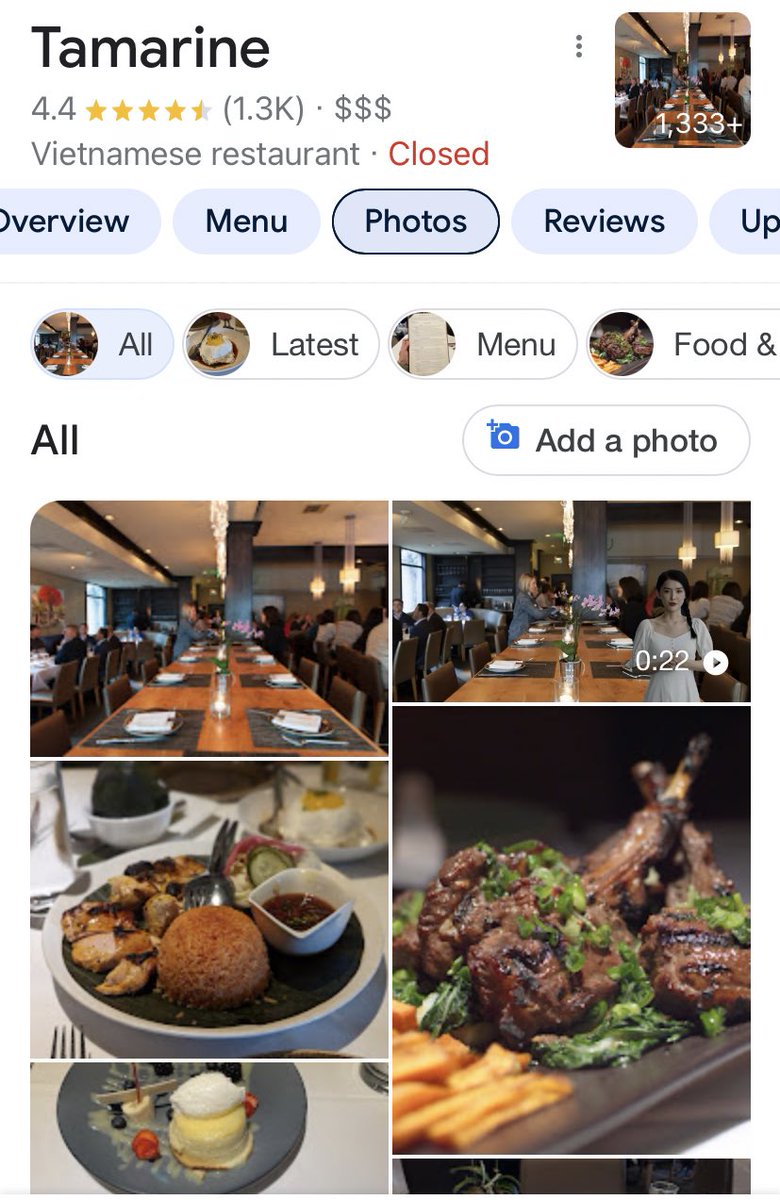**Tamarin Restaurant - Vietnamese Cuisine**

**Rating: 4.4 stars (Based on 1.3k reviews)**  
**Price: $$$**

An inviting and popular Vietnamese restaurant, Tamarin, boasts a rating of 4.4 stars from over 1,300 reviews. The ambiance is both cozy and elegant, with neatly set large tables that can accommodate groups of friends or family gatherings.

- **Table Setting:** The restaurant features large tables adorned with neatly folded napkins and clean plates, waiting to be filled with delectable Vietnamese dishes.
  
- **Food and Presentation:** 
  - A dish with a white plate elegantly arranged with a savory brown meatball, tender chicken pieces, a small cup filled with flavorful dipping sauce, freshly sliced cucumbers, and a perfectly boiled egg.
  - Another dish presented on a grey plate features a whimsical dessert with a yellow ball topped with a white sphere, garnished with a banana slice on a stick, blueberries, and a strawberry.
  - A mouth-watering grilled meat plate with finely chopped green vegetables and crispy French fries, showcasing the restaurant's versatility and finesse in both traditional and modern Vietnamese cuisine.

- **Restaurant Atmosphere:** A snapshot captures a serene table setup with no diners, accentuating the pristine and inviting dining environment. Another image highlights a woman wearing a white dress, her black ponytail draped over her left shoulder, seated at a table. In the background, other patrons can be glimpsed enjoying their time near a bar illuminated by stylish hanging lights. 

Overall, Tamarin offers a delightful dining experience with its diverse menu, meticulous presentation, and warm, inviting atmosphere. Be sure to check their latest menu, reviews, and add your own photo review after dining. 

(Note: The restaurant is currently closed but check back for updated hours and availability.)